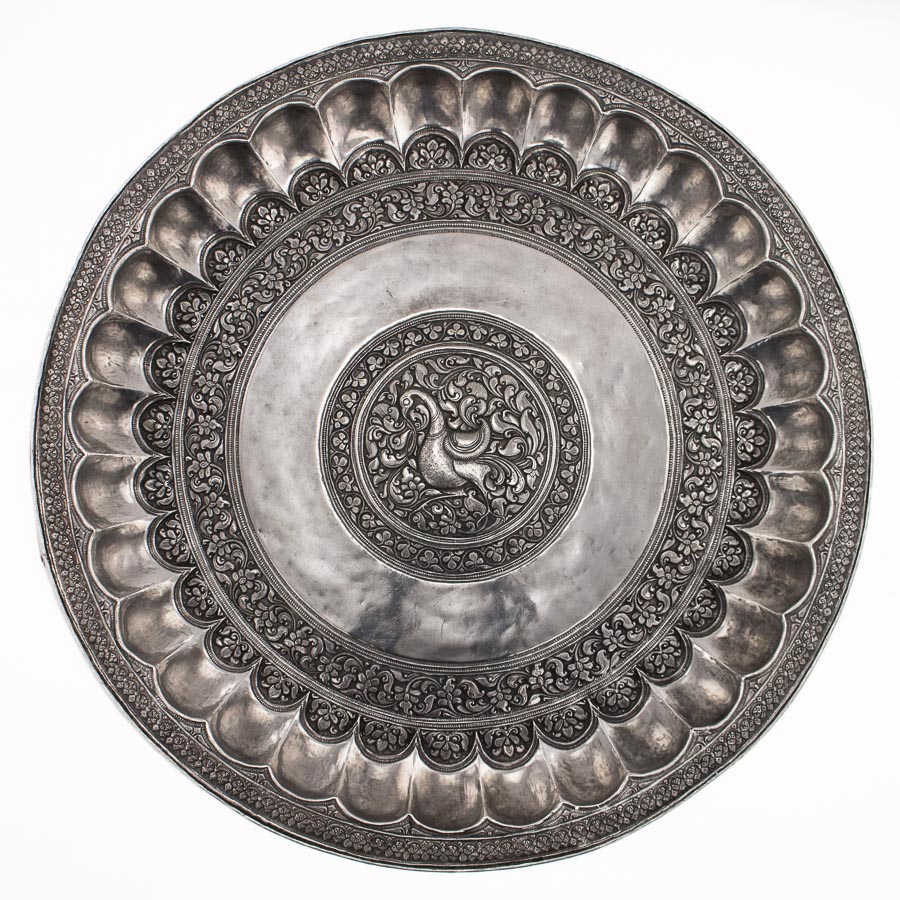This image depicts an ornate, round, silver-toned metallic piece, possibly a platter or a plaque, displaying signs of age with a somewhat tarnished and burnished appearance. The circular object, resembling a large coin or elaborate pendant, is intricately designed with at least ten distinct concentric rings. Each ring varies in width and showcases different patterns, resembling shells or Fibonacci sequences, contributing to the piece's intricate texture.

At the very center of the piece is a large circle, which hosts a detailed and stylized depiction of a bird, possibly a goose, standing with flowing tail feathers intertwined with surrounding flowers. This central motif is bordered by several layers of elaborate designs: starting with smaller rings featuring motifs that include garlands of flowers, scalloped floral patterns, and potentially three-leaf clovers. Proceeding towards the outer edge, the designs continue with ornamental detailing and small dot patterns, adding to the overall ornate aesthetic of the piece. The absence of a background in the image emphasizes the artistic workmanship and historical essence of this elaborate metallic artifact.